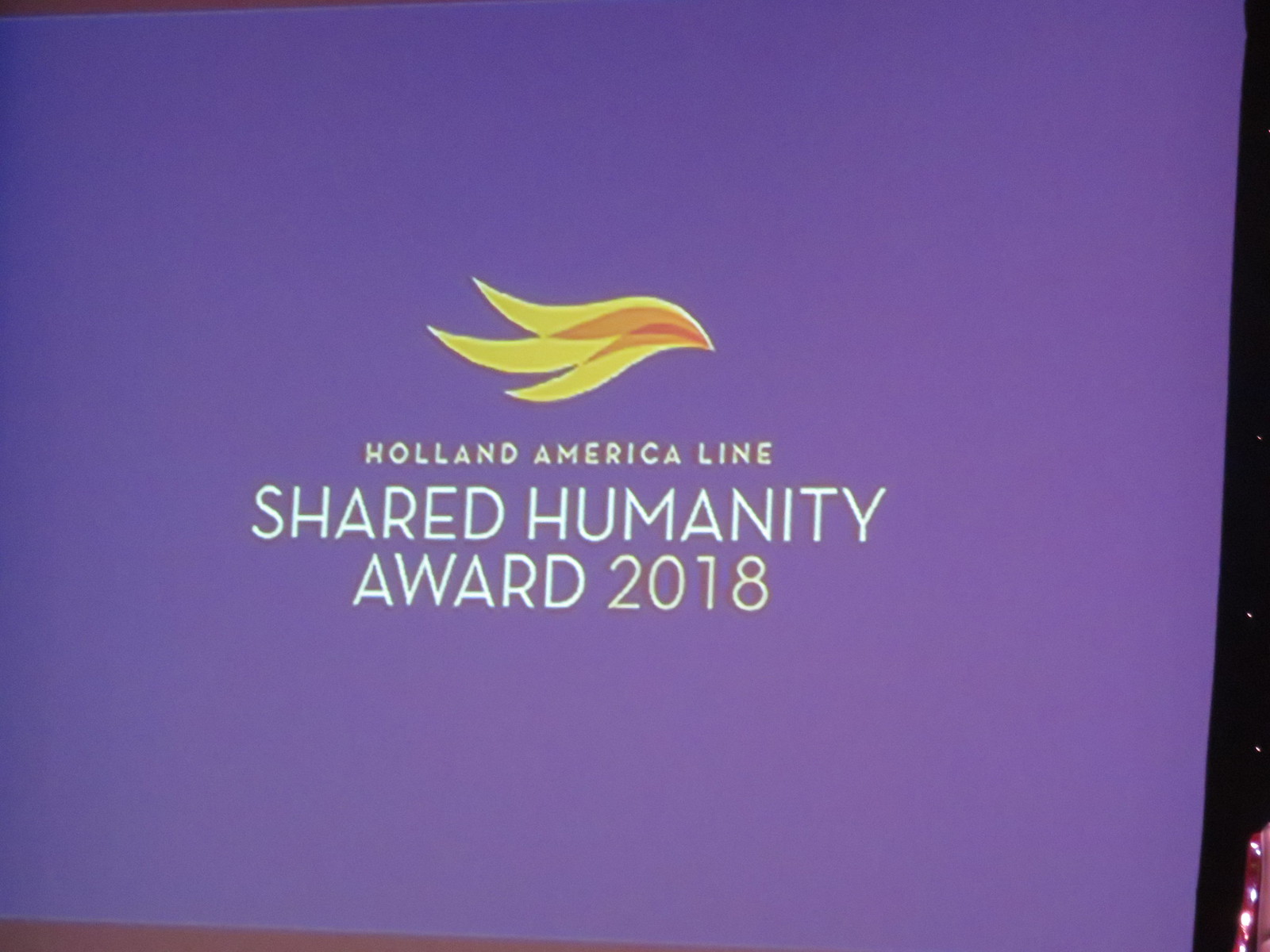The image depicts a large sign with a purple background, prominently featuring the text "Holland America Line Shared Humanity Award 2018" in white lettering. Centered above the text is a substantial yellow and orange wavy logo, potentially resembling a flame. The sign's configuration suggests it could be a banner, placard, or screen projection, though its exact size remains uncertain. The edges of the purple background transition to black on the right side, hinting at an open space or possibly a reflection, though the details are indistinct. The high contrast of the white text against the purple makes the wording clear and easy to read. The image lacks additional context or surrounding elements, focusing solely on the sign itself.